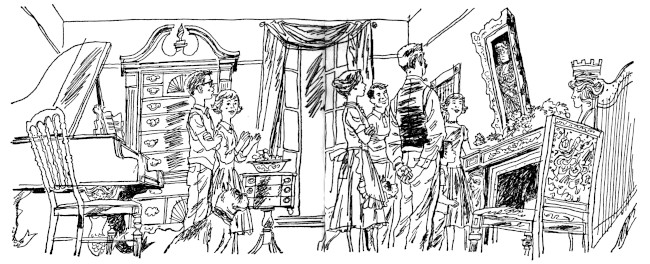In this black and white sketch drawing, a family gathers in a spacious, well-lit room dominated by whites and blacks. At the center of attention is a portrait with a female figure, likely the family matriarch, hanging over a white fireplace adorned with intricate details and accented by black interior. The top of the portrait leans slightly outward from the wall. The room features a large, open window with draped curtains, which floods the scene with light. Next to the window stands a large dresser with a carved candle on top. 

The family members are dressed in period clothing: the women wear dresses, with older women in floor-length gowns and a young girl in a knee-length dress. The men don long-sleeve shirts and trousers, while there is a boy in short-sleeve attire. A dog sits comfortably beside the boy. 

Furniture in the room includes a piano situated to the left, with a chair placed at its side. A smaller cabinet stands in front of the window, holding a bowl on top. Additional chairs are scattered around, providing seating for the family. Notably, there is a person wearing a crown near a harp on the right side, adding a touch of regal flair. The walls are white with black trim, and a horizontal strip runs around the room, tying together its classic, cohesive design.